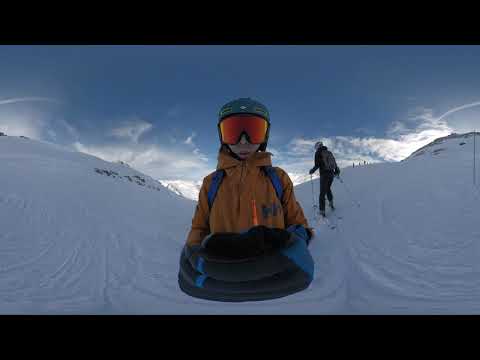The image depicts a manipulated, snowy outdoor scene set under a cloudy blue sky. Predominantly in the center is a person clad in an orange jacket and orange-lensed ski goggles, seemingly positioned in a sled or tube, although their legs and feet are not visible, suggesting manipulation. The individual appears to have blue and black gloves on their clasped hands. To the right, in the background, is another person using skis, moving in a slightly backward diagonal direction. The ground and hills are blanketed in snow, surrounded by smoke-like clouds, creating a dynamic atmosphere. The entire image is framed by a solid black border, highlighting the snow-covered landscape and emphasizing its midday setting on what could be a sledding hill.